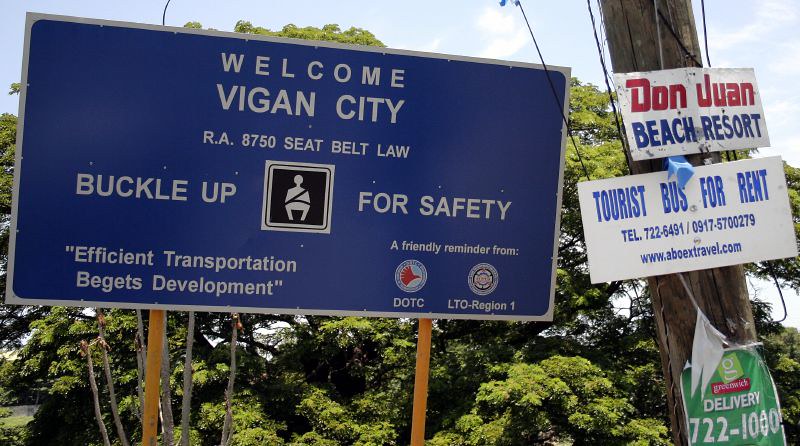The photograph is a full-color outdoor image captured on a clear summer day under a light blue sky with a few scattered white clouds. The background is dominated by lush, green leafy trees, creating a serene, natural setting. Central to the scene is a large blue rectangular street sign mounted on two wooden posts. In bold white text, the sign prominently reads:

"Welcome Vigan City RA 8750 Seatbelt Law 
Buckle Up for Safety"

Between the phrases "Buckle Up" and "for Safety," there is a logo featuring a stick figure wearing a seatbelt. Below this, in italicized white font, the sign also states:

"Efficient Transportation Begets Development"

Additionally, it bears a friendly reminder from the "DOTC LTO Region 1." To the right of this large sign, a telephone pole extends upwards, attached to which are three smaller signs. The top sign advertises "Don Juan Beach Resort," below it is a sign offering "Tourist Bus for Rent" along with contact details and a website, and the bottom green sign advertises "Greenwich Delivery" with a contact number.